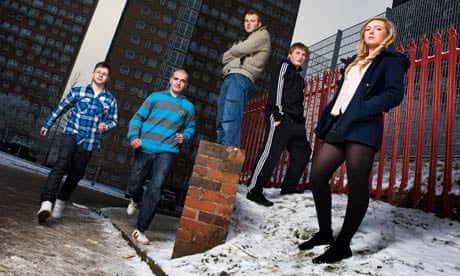In this mid-2000s album cover-esque photograph, five young individuals, likely in their late teens or early 20s, are captured in a cityscape with a light dusting of snow on the ground. To the left, two men walk forward: the first man wears a blue and white flannel plaid shirt with black jeans and white shoes, while the second man sports a blue and gray striped long-sleeved top paired with blue jeans and white shoes. In the center of the image, a man stands confidently atop a three-foot-high red brick structure, his arms crossed, wearing a gray jacket and blue jeans. To his right stands another man in a black tracksuit with white stripes, hands in his pockets. On the far right, a blonde woman dressed in a navy suit jacket and shorts, with a white shirt and tights, completes the group. They stand in front of two high-rise apartment buildings with a red slatted fence to the right and a grassy area covered in light snow to the left. The scene blends the urban environment with personal styles that reflect a bygone era.